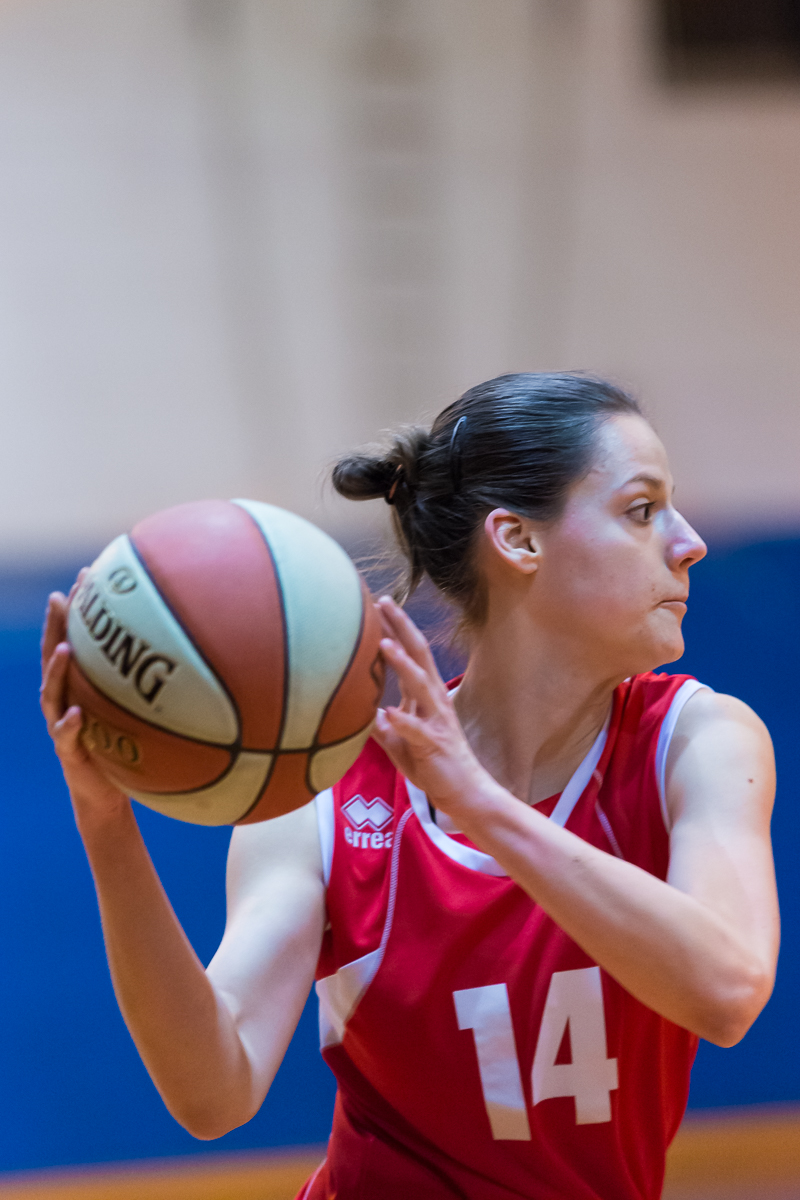The image captures a close-up view of a female basketball player with a focused expression, her body facing the camera but her head turned to the right, eyes wide open as if scanning for a teammate. She is holding a Spalding basketball, which features a mix of red, yellow, and white blocks. The player, whose dark hair is pulled back into a braided bun secured with black clips, wears a sleeveless red jersey with white stripes and the number 14 emblazoned on the chest. On the top left shoulder of her jersey, there is a logo consisting of two overlapping squares with partially visible letters "E-R-R-E" beneath it. The background is a bit blurred, featuring a white upper section and a blue lower section, with a faint gray area suggesting a pennant or similar object. In the top right corner of the image, a small black box, possibly part of a scoreboard, is visible.